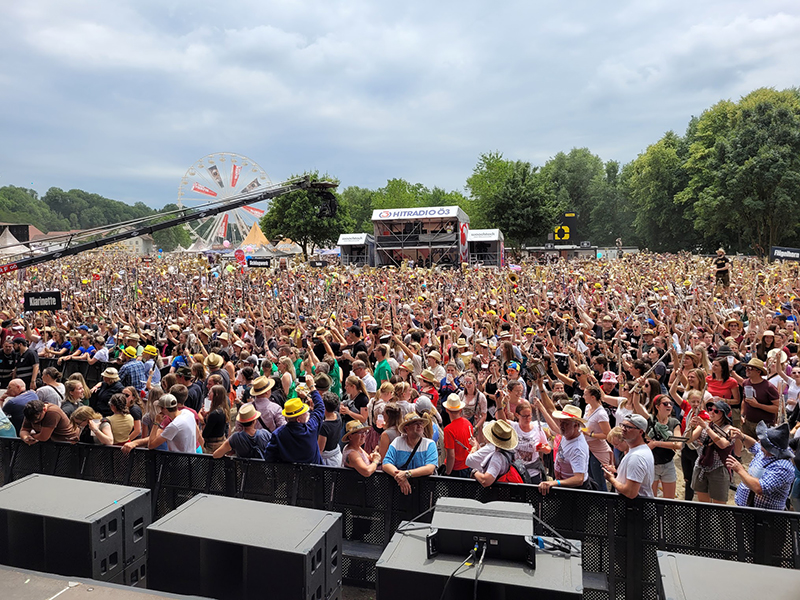This color photograph captures a vibrant outdoor event at what appears to be a fairgrounds or concert venue. The view is from a stage looking out into a massive crowd, notably composed of several hundred to possibly thousands of people dressed in bright summer clothing, with many wearing hats and short sleeves. The crowd is densely packed, pressing up against a black metal-grilled barrier that separates them from the stage area. On this side of the barrier, there are numerous black cubical metal structures, likely electronic devices or amplifiers for a concert. In the background, a Ferris wheel towers above a series of tent pavilions. A two-story building with an open front prominently displays the sign "Hit Radio 03" across its roof. Green trees create a scenic horizon against a blue sky scattered with white clouds. Additionally, a crane extends over the crowd to the left, adding to the bustling atmosphere of the scene.